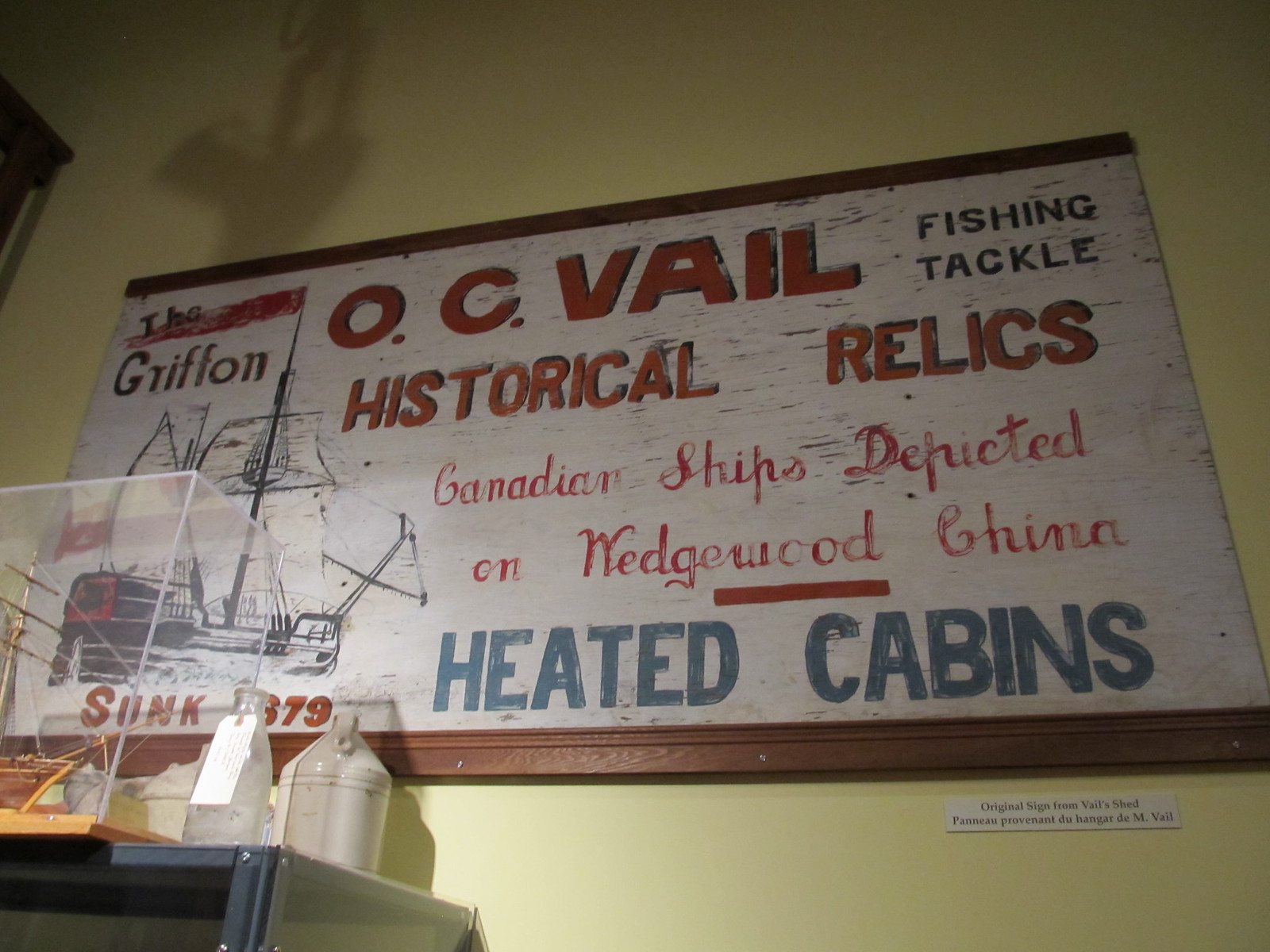The image is a photograph taken inside a museum, showing a long, horizontal, rectangle-shaped sign fixed on a yellow wall. The sign has a wooden frame at the top and bottom, both painted maroon. At the top in maroon letters, it reads "O.C. Vale Historical Relics." Just below, in maroon script, it says "Canadian Ships Depicted on Wedgwood China." To the right, in black letters, it states "Fishing Tackle." Prominently centered at the bottom in all caps blue letters, it announces "HEATED CABINS." 

On the left side of the sign, there is a detailed sketch of a sailing vessel with at least three sails. A maroon flag with the name "The Griffin" is flown from the ship. Underneath the name, the word "sunk" is written, followed by barely visible numbers ending in "79."

Underneath the sign, there is a plexiglass enclosure holding a model of a sailing ship, most likely a Three-Master, although only the front end is visible. Next to the model ship, a few old whiskey jugs are placed, adding to the antique ambiance of the display.